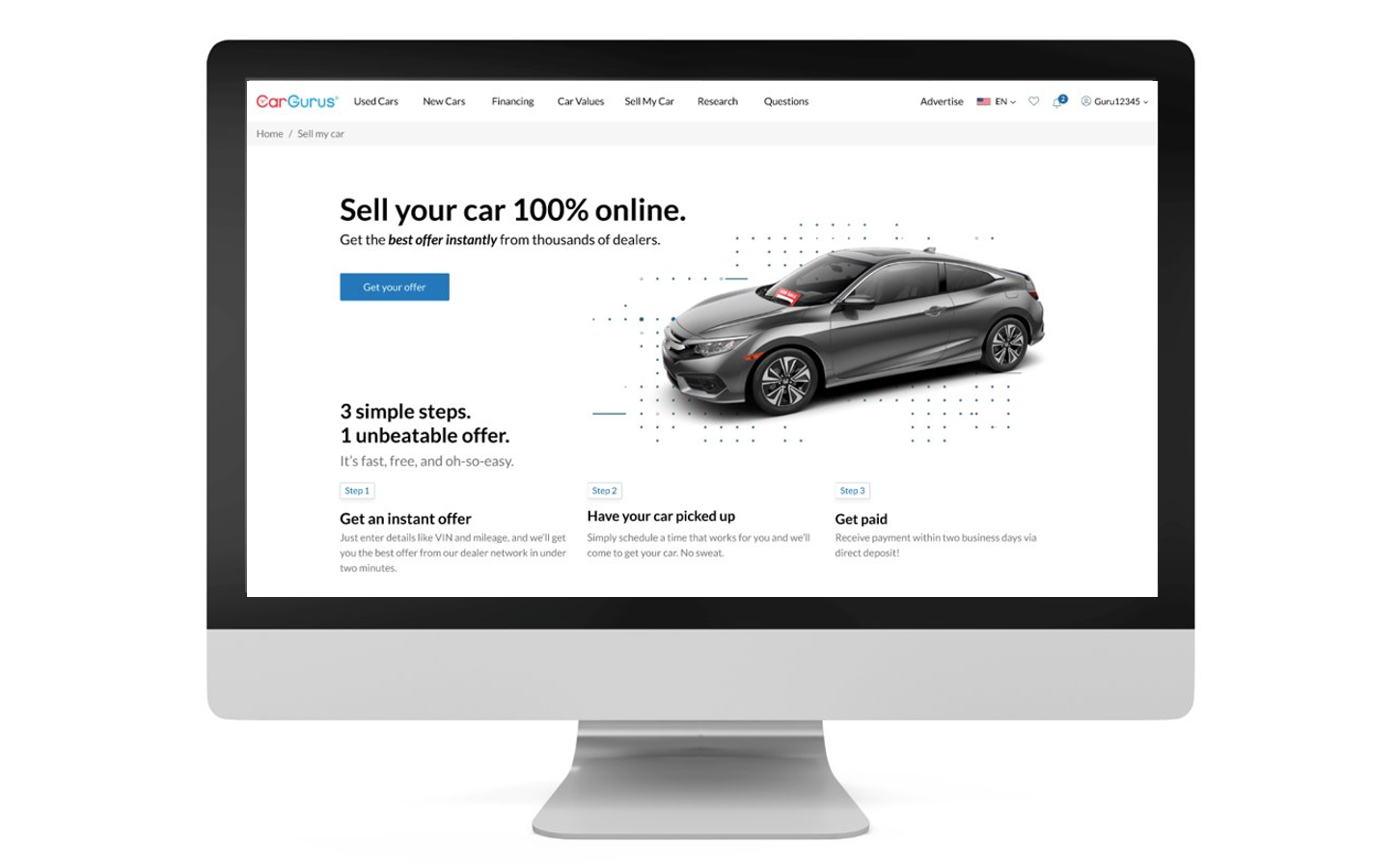The image depicts an Apple all-in-one computer, prominently featuring a sleek monitor with black bezels and a signature Apple silver base. The monitor displays the CarGurus website, which is advertising its service of selling cars 100% online. A central image on the website shows a silver sedan, complemented by the text, "Get the best offer instantly from thousands of dealers. Get your offer." The site also highlights a navigation bar with categories such as "Used Cars," "New Cars," "Financing," "Car Values," and "Sell My Car." Additionally, a section on the website promotes the simplicity of their service with the phrase "Three simple steps, one unbeatable offer." The overall impression of the website is that of a corporate platform designed to facilitate car sales. It remains unclear whether the image's purpose is to promote CarGurus, the Apple computer, or both.